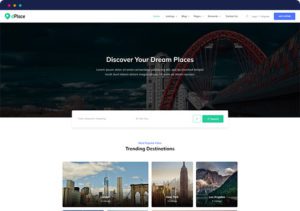A detailed caption for the described image could be:

"This image appears to be a screenshot from a Mac computer, displaying a city-themed webpage. At the top left, it has the characteristic red, yellow, and green dots typical of a Mac window. Below these, there is a green pin icon indicating a location on a map, followed by partially legible text. Underneath a blue navigation bar with about six or seven clickable buttons is another blue button labeled 'Discover Your Dream Place,' accompanied by an unreadable description. The background behind the buttons is dark, portraying a city skyline that possibly features a roller coaster with a red rail system in the foreground. Lower on the page is a search box with two input fields, a drop-down menu, and a green button. Below the search function, there are three cityscape images: the first shows skyscrapers and clouds, the second is a close-up of a needle-like skyscraper suggesting it might be New York City, and the third features a scenic nature view. Above these images, blue text includes a partially readable phrase 'Trending Destinations,' highlighting popular city and nature destinations."